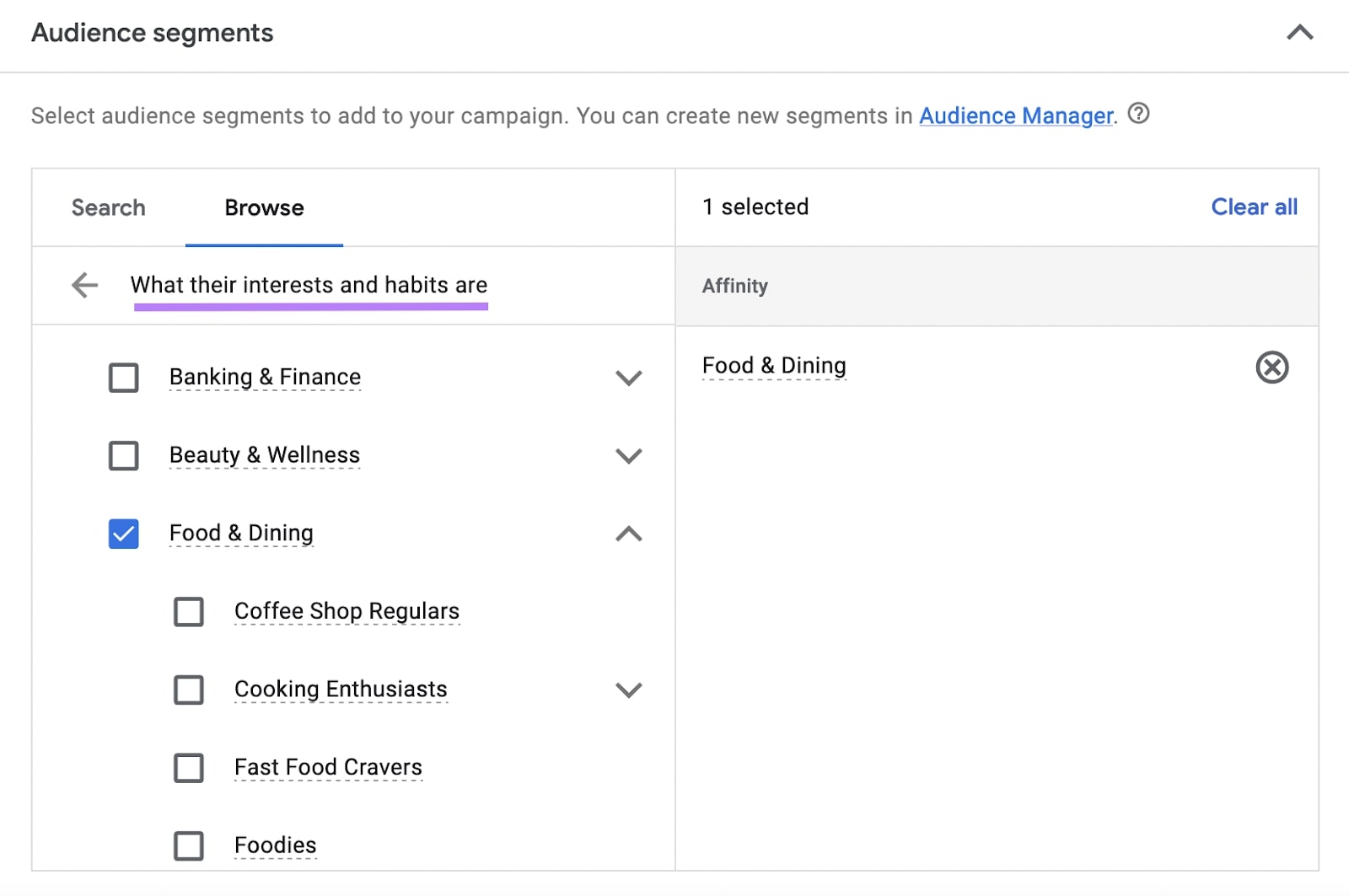At the very top of the image, bold black text reads "Audience Segments," with a horizontal line below it. Underneath, it says, "Select audience segments to add to your campaign." The phrase "You can create new segments in Audience Manager" is highlighted in blue and underlined. 

Below this, there are two tabs: "Search" in black text on the left, and "Browse" in blue, underlined text on the right. Below these tabs, a left-pointing arrow is present next to the phrase "What their interests and habits are," which is underlined in a thick purple line.

A list of options follows, marked by small squares:
1. Banking and Finance
2. Beauty and Wellness
3. Food and Dining (this square is filled in blue with a check mark inside)
4. Coffee Shop Regulars
5. Cooking Enthusiasts
6. Fast Food Cravers
7. Foodies

To the right, it states "1 Selected," with an option to "Clear All" next to it. Below this is a long gray box containing the word "Affinity."

Underneath, "Food and Dining" appears in black text, underlined with broken lines. To the right of this option is the symbol to remove it: an 'X' inside a circle.